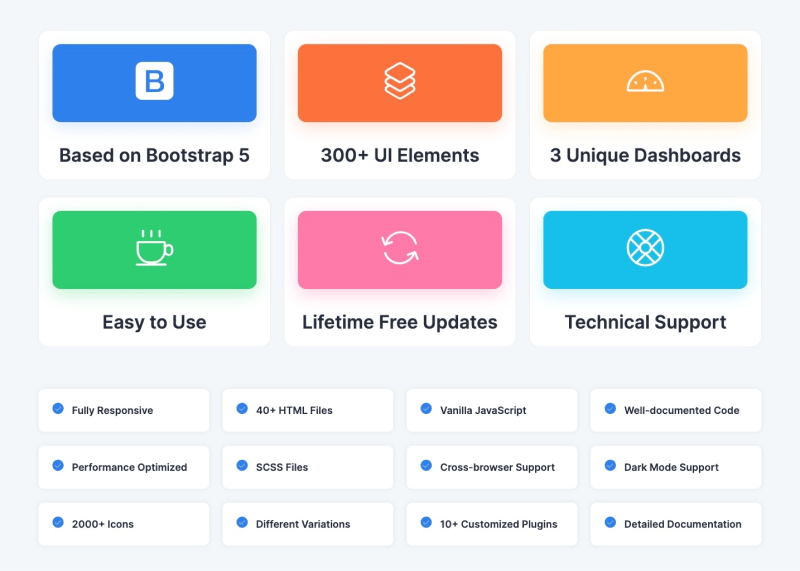This image depicts a computer screen showcasing a webpage. At the top, there are six colorful square icons, each representing different features:

1. In the upper-left corner, a blue box contains a white square with a blue letter "B" inside, indicating the page is based on Bootstrap 5.
2. To the right, an orange box features stacked squares with the text "300+ UI elements."
3. Next, a golden-yellow box shows a timer icon and proclaims "3 unique dashboards."

Dropping down to the next row:
4. A green box with a steaming coffee cup signifies "easy to use."
5. In the middle, a pink box with two circular arrows promises "lifetime free updates."
6. Lastly, a teal box with an "X" symbol offers "technical support."

Below these icons, there are three additional rows with four sections each, characterized by clickable dots, indicating further interactive areas or options. The overall design is visually systematic, highlighting various functional aspects with distinct icons and colors.